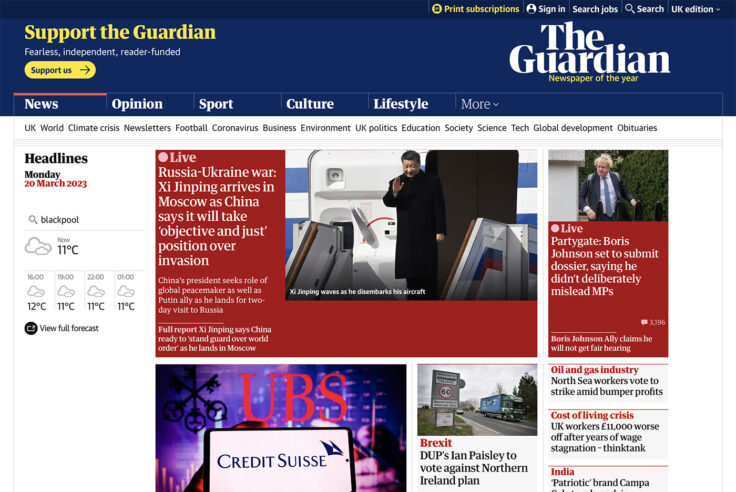Here is a detailed caption based on the provided information:

---

**Port the Guardian | News, Opium, Sport, Culture, Lifestyle**

**Headlines: Live Russia-Ukraine War**

- **Xi Jinping's Moscow Visit:** Xi Jinping has arrived in Moscow as China's diplomatic stance evolves. China has announced its intention to adopt an "objective and just" position regarding the ongoing Russia-Ukraine invasion.
  
- **Partygate Scandal:** Boris Johnson is preparing to submit a comprehensive dossier aiming to prove that he did not intentionally mislead Members of Parliament (MPs) during the Partygate scandal, which has caused significant political turmoil.

- **UBS and Suicide:** In a shocking turn of events, UBS credit is connected to a suicide case, stirring emotional and legal ramifications.

- **Northern Ireland Plan:** Democratic Unionist Party (DUP) member Ian Paisley is set to vote against the proposed Northern Ireland plan.

- **North Sea Workers' Strike:** Workers from the oil and gas industry in the North Sea have voted to strike, highlighting ongoing labor disputes and issues surrounding industry profits.

- **UK Cost-of-Living Crisis:** A think tank report has revealed that UK workers are now £31,000 worse off after years of wage stagnation, exacerbating the cost-of-living crisis.

- **Indian Brand Campa:** In alignment with national pride, India promotes the patriotic brand Campa, which is becoming increasingly popular among consumers.

---

This caption provides a comprehensive summary of the key points mentioned in the original, focusing on clarity, detail, and readability.